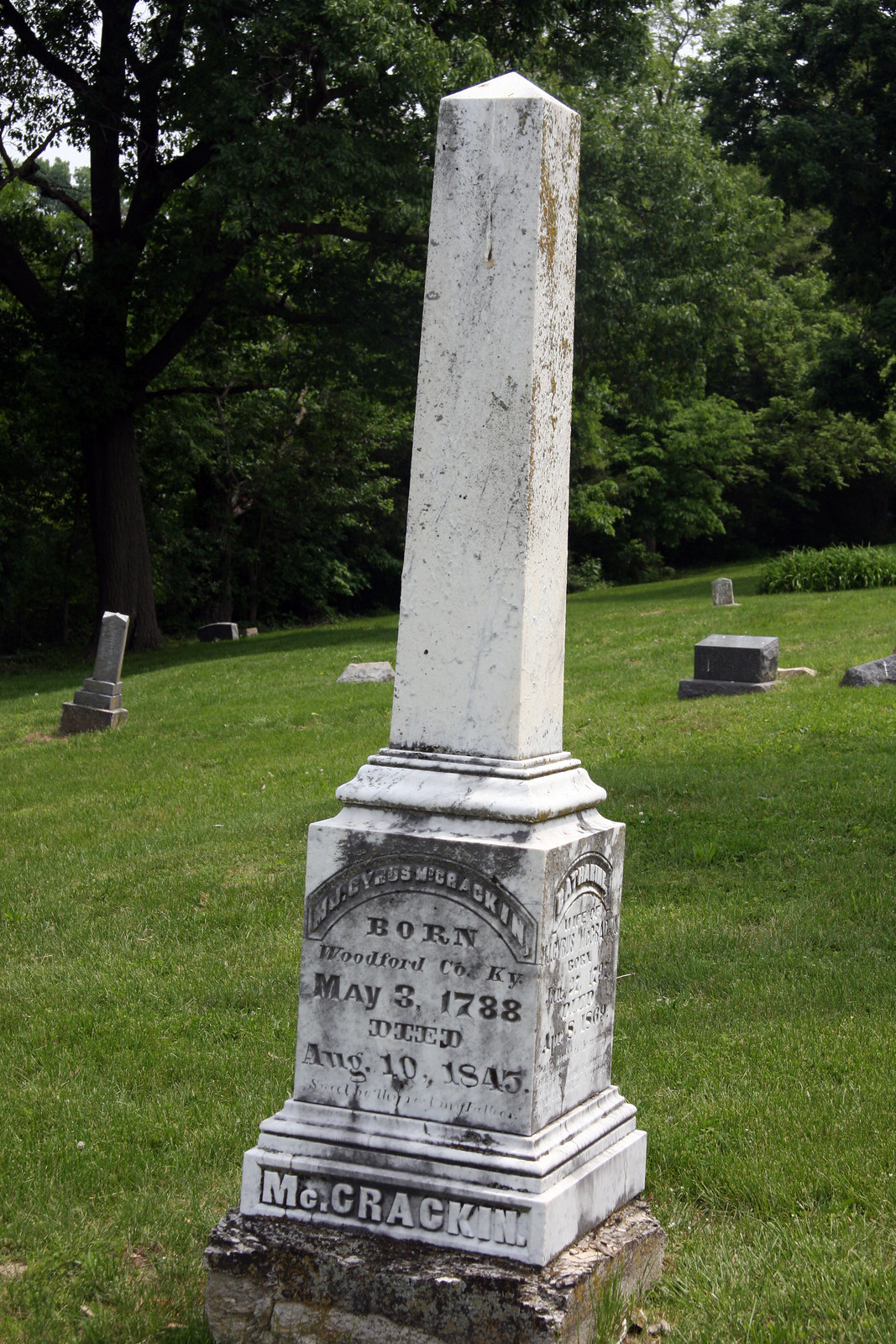The photograph, taken in portrait mode during the daytime, depicts a serene cemetery scene dominated by a tall, white gravestone resembling the Washington Monument. The gravestone, made of cement and tinged with grime, stands prominently in a lush, grassy field. The stone features an inscribed archway on its wider base that reads "MJ Cyrus McCracken" and a partially visible name "Catherine" on the right, likely obscured by dirt. The primary inscription, "Born Woodford County, Kentucky May 3rd, 1788" and "Died August 10th, 1845," marks the lower third of the monument. At the very bottom, "McCracken" is distinctly carved in capital letters with a period. Surrounding the central gravestone are smaller gravestones scattered throughout the grassy expanse. The background of the photograph is filled with dense green trees, with bits of blue sky peeking through the foliage, adding a peaceful, wooded backdrop to the cemetery scene.